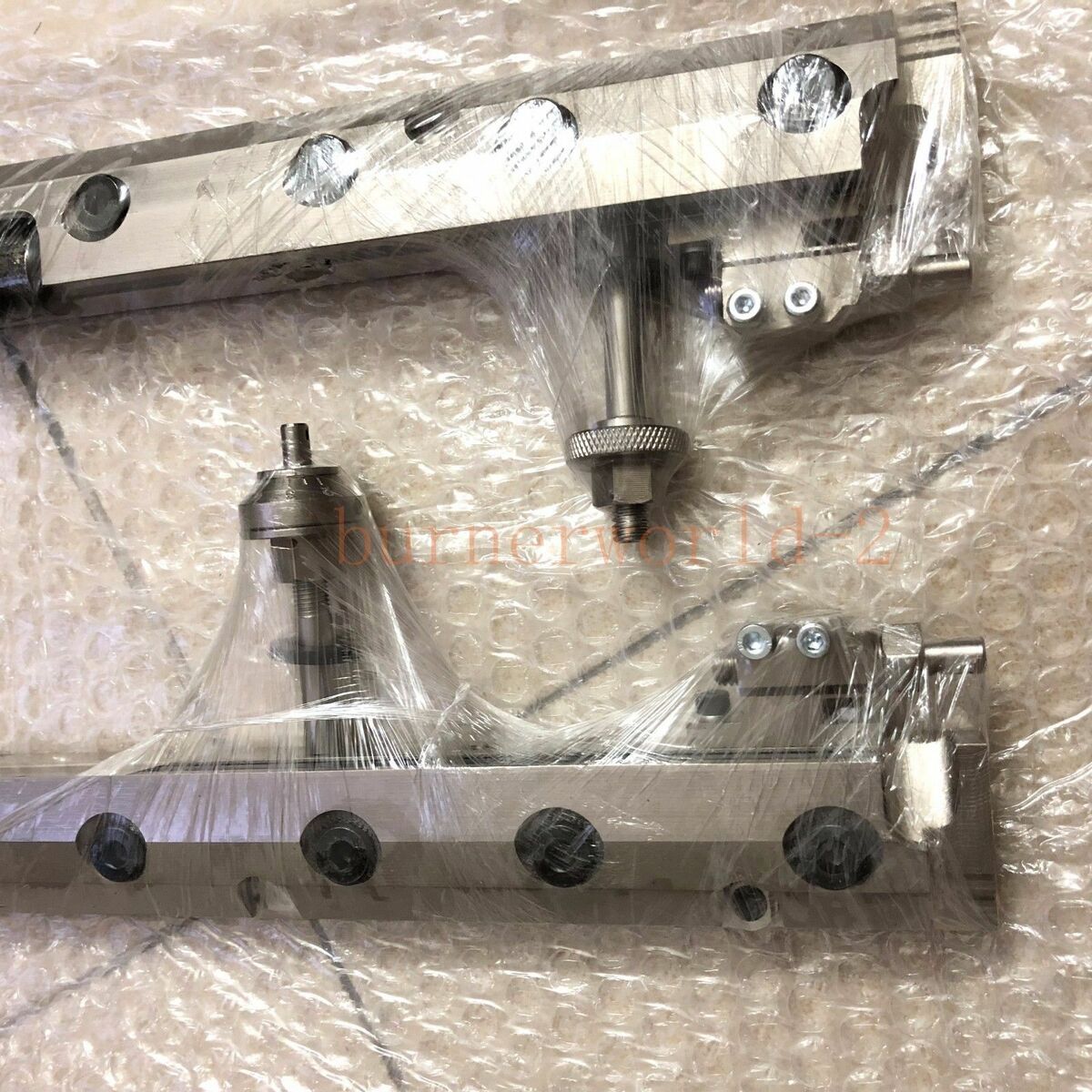The photograph depicts two wrapped metallic tools displayed on a clear bubble wrap sheet against a fluorescent square-tiled floor. Both tools are similarly shaped, resembling an elongated 'L', with a large post topped by a knob positioned at their midsection. These metal parts, secured in shrink wrap and possibly vacuum-sealed, exhibit four prominent circles along their lengths, which could be described as bolts or screw fixings. Although a portion of the bubble wrap appears deflated or popped, the shrink wrap around the tools has been meticulously applied, though one tool shows a tear on the left side where the protective wrap is absent. The metallic surfaces of the tools exhibit an assortment of colors including silver, brown, and black circular features, potentially hinting at wheels. The tools seem to rest upon bubble wrap not entirely contained, suggesting recent handling or unwrapping. A faint, unreadable pale pink watermark on the floor adds an additional layer of detail to the scene. One tool lies upside down and reversed, whereas the other stands upright beside it.